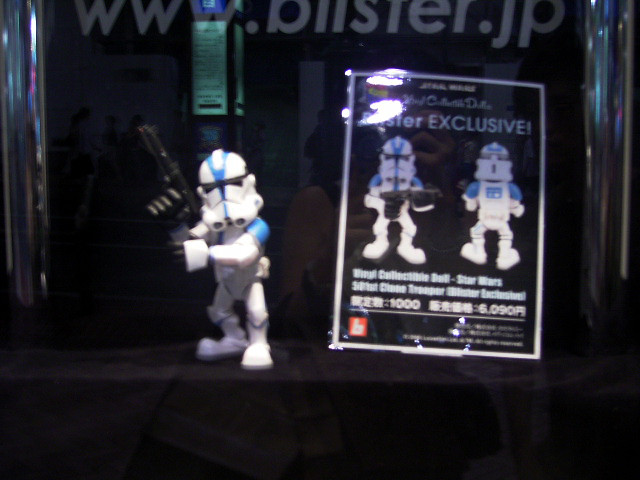The image depicts a detailed and intricately displayed collectible figurine of a Star Wars clone trooper, positioned in a display case. The trooper, primarily white with blue accents on the center of the helmet and shoulders, stands to the left of center within the case. The figure is wielding a black gun in its right hand and is situated on a black surface and background, likely a black tablecloth or blanket. The trooper's stance features the right foot turned to the left and the left foot pointing forward, and it sports a characteristic black visor across the eyes.

Adjacent to the trooper on the right is a black poster that reinforces the exclusivity of the display. The poster features two images of similar action figures, the first holding a gun and the second unarmed. Above these images, in slightly unclear text, the word "exclusive" can be prominently read. The bottom corner of the poster flaunts a distinctive red emblem, with additional lines of white print within the frame, somewhat blurred. At the top of the poster, a website URL partially visible as www.something.jp extends off the image.

The display case itself is notable for its reflective glass surface, which reveals the reflections of people and various elements within the surrounding environment, including what appears to be a pillar with a sign and additional people. The exterior of the photograph is framed by silver cylindrical pillars, enhancing the overall sophisticated presentation of this collectible trooper figure.